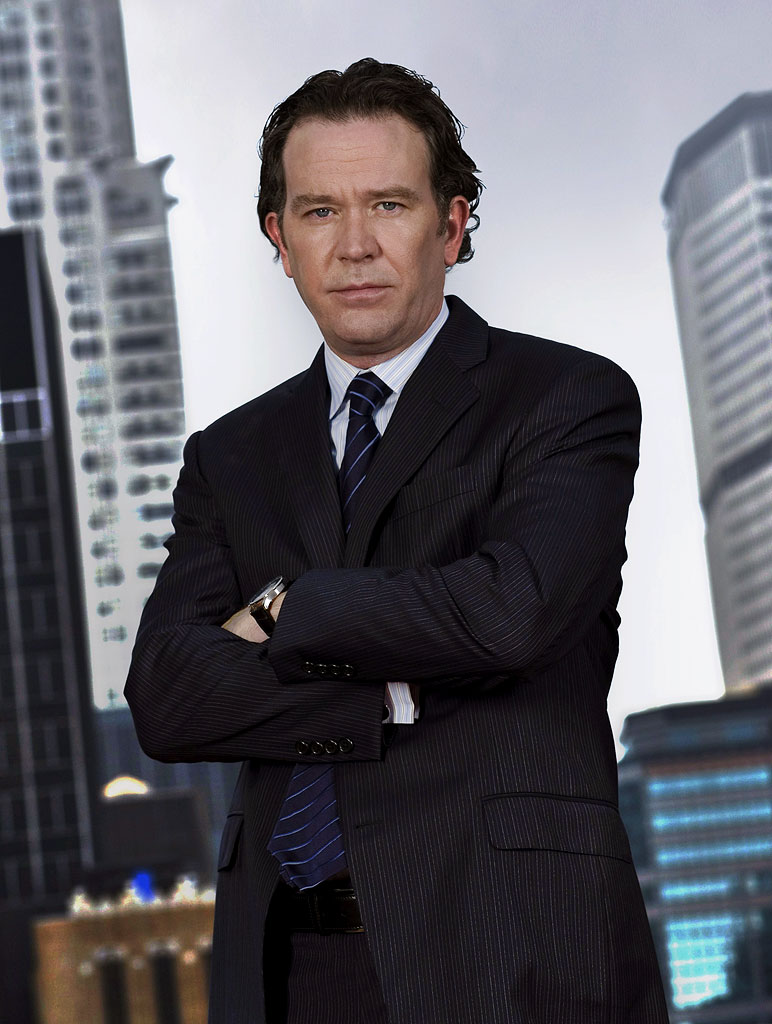In this photograph, actor Tim Robbins stands centrally, clad in an elaborate black and white pinstriped suit jacket over a white dress shirt, complemented by a blue tie with diagonal stripes and a mix of white and blue crosses. His neatly slicked-back dark brown hair frames his neutral facial expression as he looks directly into the camera. His arms are folded, revealing a wristwatch on his left wrist with a slender leather band and a silver frame. Behind him, an array of skyscrapers and high-rises appear, likely forming part of a city skyline, though it gives the impression of being an indoor setting with a backdrop featuring buildings in black, silver, brown, and blue hues, set against a predominantly white and gray sky. The ensemble and the urban backdrop suggest a polished and sophisticated portrayal of the actor.